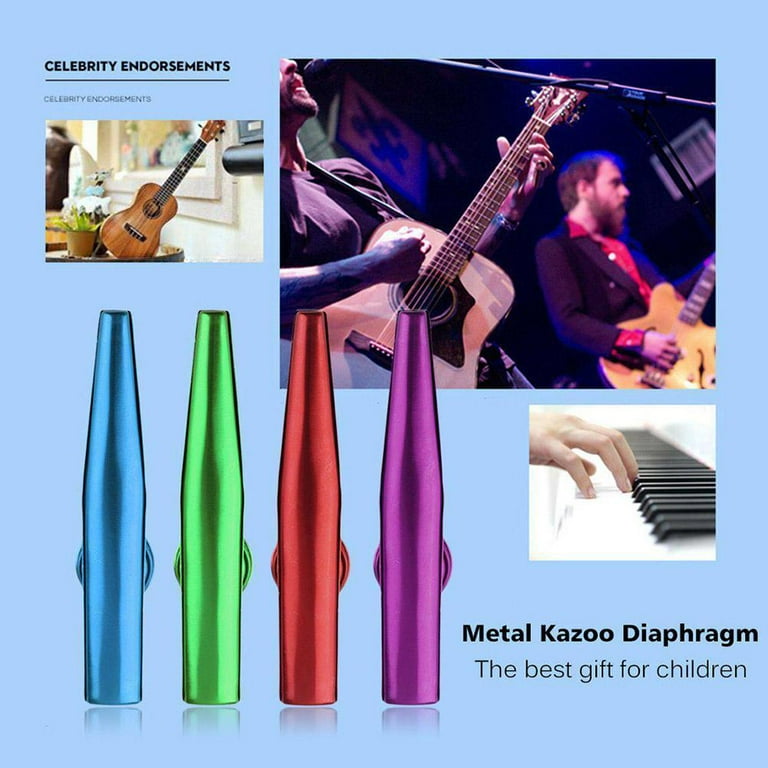The image features a vibrant display of metal kazoos in blue, green, red, and purple, each with a cylindrical bottom and tapered top. Accompanying black text labels these as "metal kazoo diaphragm" and describes them as "the best gift for children." Surrounding this central theme, a collage of stock images on a baby blue background showcases various musical elements: a hand playing piano keys, two men engaged with guitars—one on an acoustic guitar, the other on an electric guitar—and another acoustic guitar near a flower pot. Above these images is bold text, underlined, stating "celebrity endorsements," though no specific endorsements appear visible. The diverse array of musical instruments hints at a broader musical theme, although their direct connection to the kazoos is not explicitly clear.